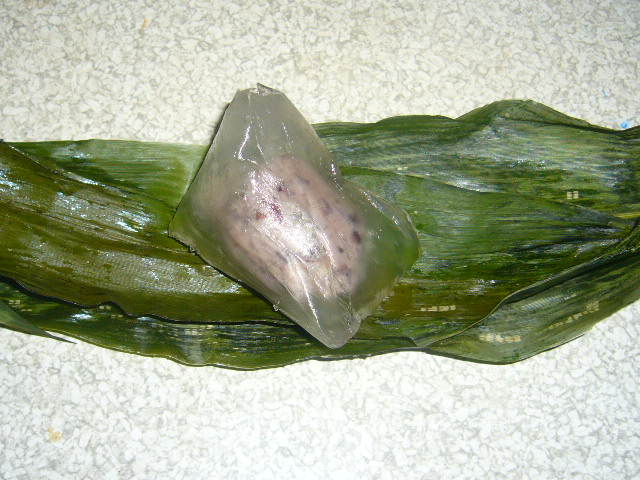The image depicts a vibrant, indoor setting, perhaps a kitchen or restaurant, featuring a centerpiece arrangement. A large, wet leaf reminiscent of a banana leaf or corn husk sprawls across the middle of the image, its slimy texture captured in various shades of green. Atop this leaf lies an unusual object that initially appears to resemble a brain or a cream-colored, spotted quail egg, encased in a clear, gelatinous bag. This enigmatic object sits precisely at the center of the frame, drawing attention with its complex texture and peculiar form. The background is a smooth, white tiled surface with a subtle design. The entire scene is colored in a palette that includes white, gray, green, pink, and purple, creating a striking contrast that enhances the intriguing, almost surreal quality of the objects displayed.